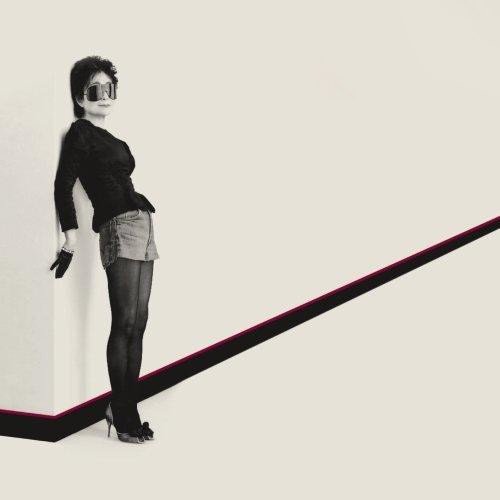The image features a woman, possibly Yoko Ono, standing against a white wall that angles close to 45 degrees. She is positioned toward the right center of the photo. This short, older-looking Asian woman wears very large polarized sunglasses that were popular in the 80s, covering her eye sockets and extending to her cheeks. Her hair is styled in a masculine haircut reminiscent of a pixie cut, suggesting a slight mohawk appearance and also typical of the 80s fashion.

Her outfit consists of high-heeled shoes with a small bow on the toe area, black leggings, jean shorts, and a black long-sleeve top that covers her entire upper torso. Her right arm, draped against the corner of the wall, is adorned with a black glove that does not quite reach her wrist. The specifics of her left arm are not visible.

She leans back slightly, with her shoulders touching the wall while her lower body remains upright and away from it. The backdrop includes a distinctive black line running along the base of the wall, with a thin red line just above it, giving the appearance of a sideways checkmark. The stark contrast of the black and white color scheme is disrupted only by this discreet red accent. Her stance and the severe minimalism of the setting create a striking, monochromatic composition.